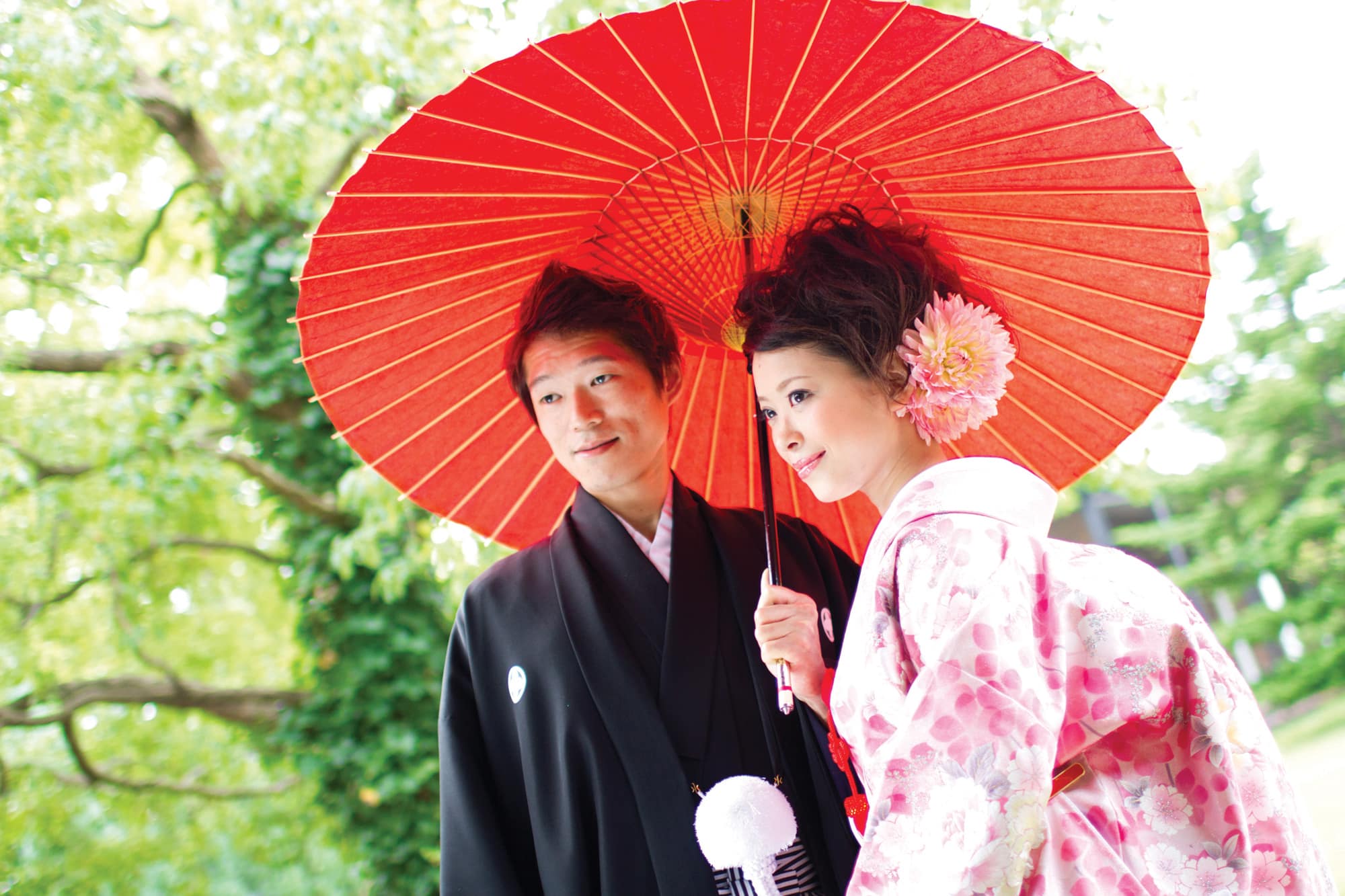In this image, a young Oriental couple, possibly of Japanese descent, is being photographed outdoors. The background is filled with lush green trees and foliage, suggesting they might be in a garden. The couple is standing tilted at an angle, approximately 30 degrees counterclockwise, giving the image a dynamic perspective. 

The male is dressed in a black kimono-like robe that resembles a tuxedo without a tie, featuring some oriental elements such as a cummerbund. He is holding a striking red umbrella with orange trim in his left hand. The female is wearing a flowing pink and white dress, possibly a kimono, adorned with floral designs. Her hair is styled in an elegant bun, accessorized with a large pink flower that matches her dress. Both of them are smiling and looking slightly to the left.

The overall composition is enhanced by the contrasting greenery in the background, which frames the couple beautifully in the bright daylight.